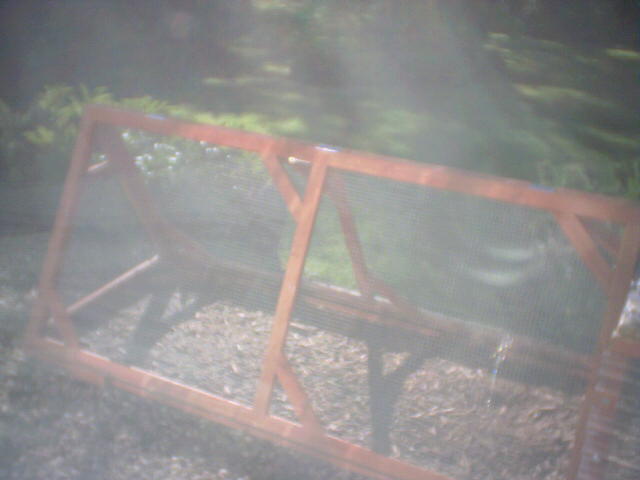This photograph captures a backyard scene featuring a chicken coop. The coop is distinctly triangular in shape, constructed with wooden supports and enclosed with mesh or wire to protect the chickens. The coop's wooden structure appears to be made from a reddish cherry wood, contributing to its rustic charm. The floor inside the coop is lined with mulch, creating a comfortable and natural environment for the chickens. On one of the panels, there is a noticeable smear of what seems to be bird droppings, indicating active use by the chickens. The background reveals a lush green yard, adorned with various bushes and trees, adding a serene, natural backdrop to the scene. The photograph, however, lacks clarity and detail, as it appears washed out, overly bright, and blurred in certain areas.